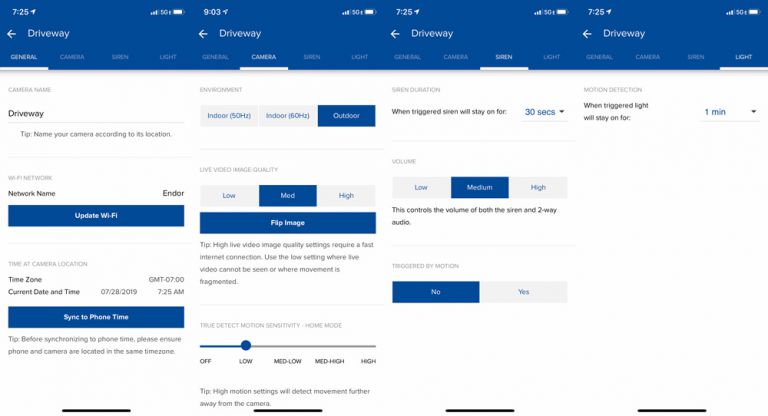This web page showcases a rather intricate interface that resembles four smartphone screens arranged side by side horizontally. At the very top, a long, horizontal blue bar spans across, featuring white text that serves a navigational or informational purpose. Each of the four "screens" displays common smartphone status icons including the time (positioned on the upper left corner), Wi-Fi signal strength, 5G connectivity, and battery levels.

Below this status bar, each screen features a left-pointing arrow beside the word "driveway," indicating that the user can navigate to a different page. The current page for all four screens is titled "driveway."

The bottom sections of three of these screens incorporate long, horizontal blue buttons with various options such as "Flip Image," "Update Wi-Fi," and "Sync to Phone Time." Additionally, one screen presents an option labeled "Triggered by Motion" with a selection of "No," and another option where "Volume" is set to "Medium."

The interface also includes tabs at the top of each screen labeled "General," "Camera," "Siren" (the third tab is slightly unclear but appears to be "Siren"), and "Light." Each screen appears to highlight a different tab, suggesting that these could be instructional panels or guides representing different features available within the same application or system. This detailed breakdown suggests that the webpage is likely an interactive display or configuration panel for some software or device.